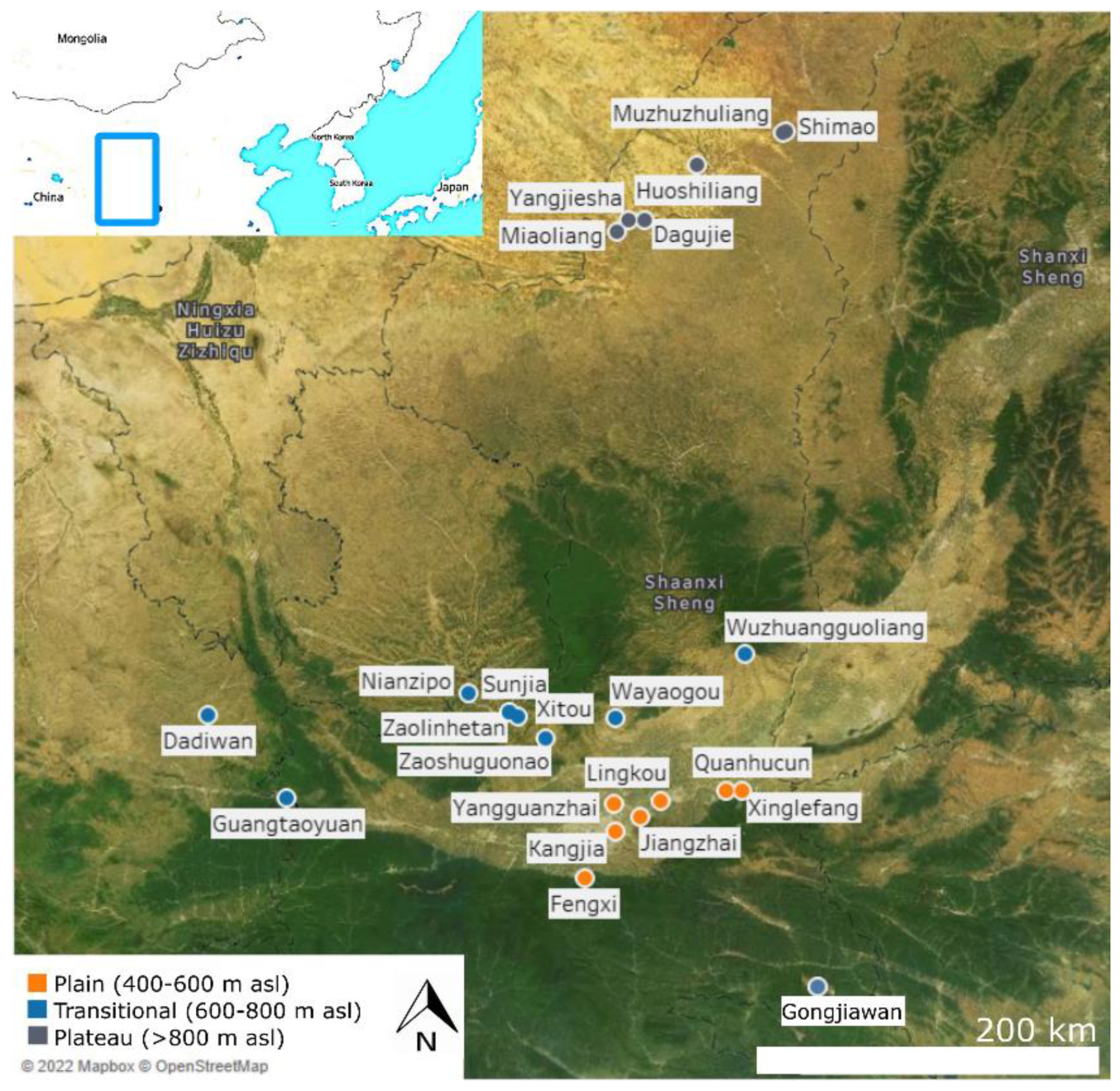This image is a detailed, edited satellite photograph of central and north-central China, annotated with various geographical and topographical information. The central focus showcases a map with distinct color zones: yellow at the top, transitioning through orange and brown, and finally green at the bottom. These colors correspond to the region's elevation levels, marked with dots and labels. Orange dots represent plains at 400-600 meters above sea level (MASL), blue dots indicate transitional areas at 600-800 meters MASL, and gray dots denote plateaus at 800 meters MASL. In the bottom left, a scale shows a white rectangle indicating 200 meters distance. The top left corner features a zoomed-out map highlighting the location within China, bordered by North Korea, South Korea, Japan, and Mongolia. The annotations and data credit Mapbox and OpenStreetMap, copyrighted in 2022.